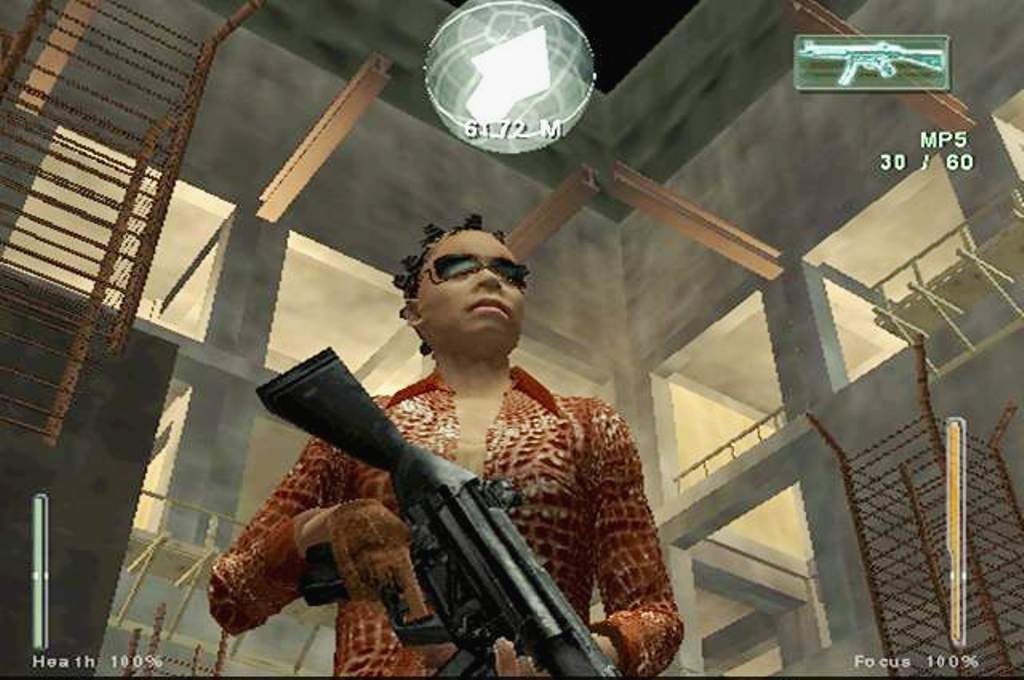A dynamic screenshot from a video game centers on the main character, who exudes a cool and edgy vibe. Sporting slick, short hair and stylish sunglasses, the character stands confident in a striking red leather jacket. He grips an MP5 submachine gun, ready for action. At the bottom left corner of the screen, the character’s health is displayed at a full 100%. The bottom right corner shows that his focus is also at 100%. The top right corner features a mini icon of the MP5 with an ammunition count of 30/60, indicating the rounds loaded and remaining. The backdrop shows an industrial grey warehouse with a set of stairs climbing upwards, contributing to the gritty, urban atmosphere of the scene.